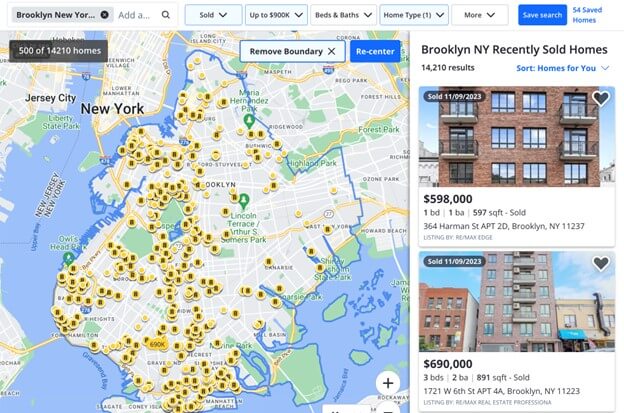The screenshot displays a detailed real estate search interface focused on Brooklyn, New York. On the left side, a map of Brooklyn is prominently featured, pinpointed with numerous yellow circles indicating the locations of properties. The map highlights the dense urban area towards the bottom left, with water bodies visible to the left, bottom, and right sides. Above the map, it is noted that 500 out of 14,210 homes are displayed.

The top left corner of the interface confirms the search location as Brooklyn, New York, while the right side of the screen showcases a list of homes that have recently been sold. Filters have been applied, including price up to $900,000, beds and baths specifications, and various home types.

Two properties are highlighted on the right side. The first is a three-story apartment building priced at $598,000, featuring one bedroom, one bathroom, and a total area of 597 square feet. The second property listed is also an apartment building, sold for $690,000, offering three bedrooms, two bathrooms, and an area of 891 square feet. Both properties are in Brooklyn, New York. The interface indicates a total of 14,210 results for recently sold homes in the area.